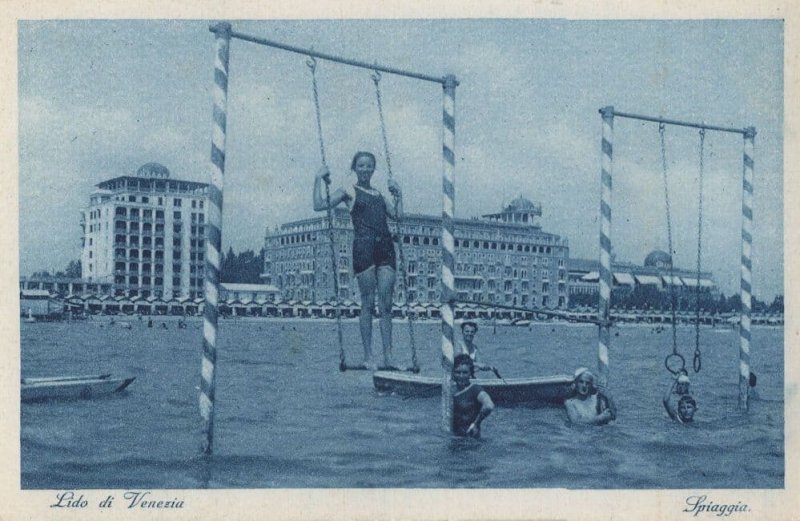This old, black-and-white photograph, which may have a postcard-like quality due to its white border, showcases a lively scene at Lido di Venezia. The image captures a group of people in the water, engaging with gymnastic equipment. Notably, two sets of tall, striped poles rise from the water, each connected by a bar at the top. On the left set of poles, a woman in a swimsuit is standing on what appears to be a trapeze-like bar, while the right set features two chains with handholds, resembling gymnastic rings. The photograph has a bluish or tan tint and feels quite vintage. Texts in cursive reading "Lido di Venezia" and "Spiaggia" are present on the bottom left and right corners, respectively. In the background, numerous small boats float near a shoreline that is lined with buildings, under an overcast sky.